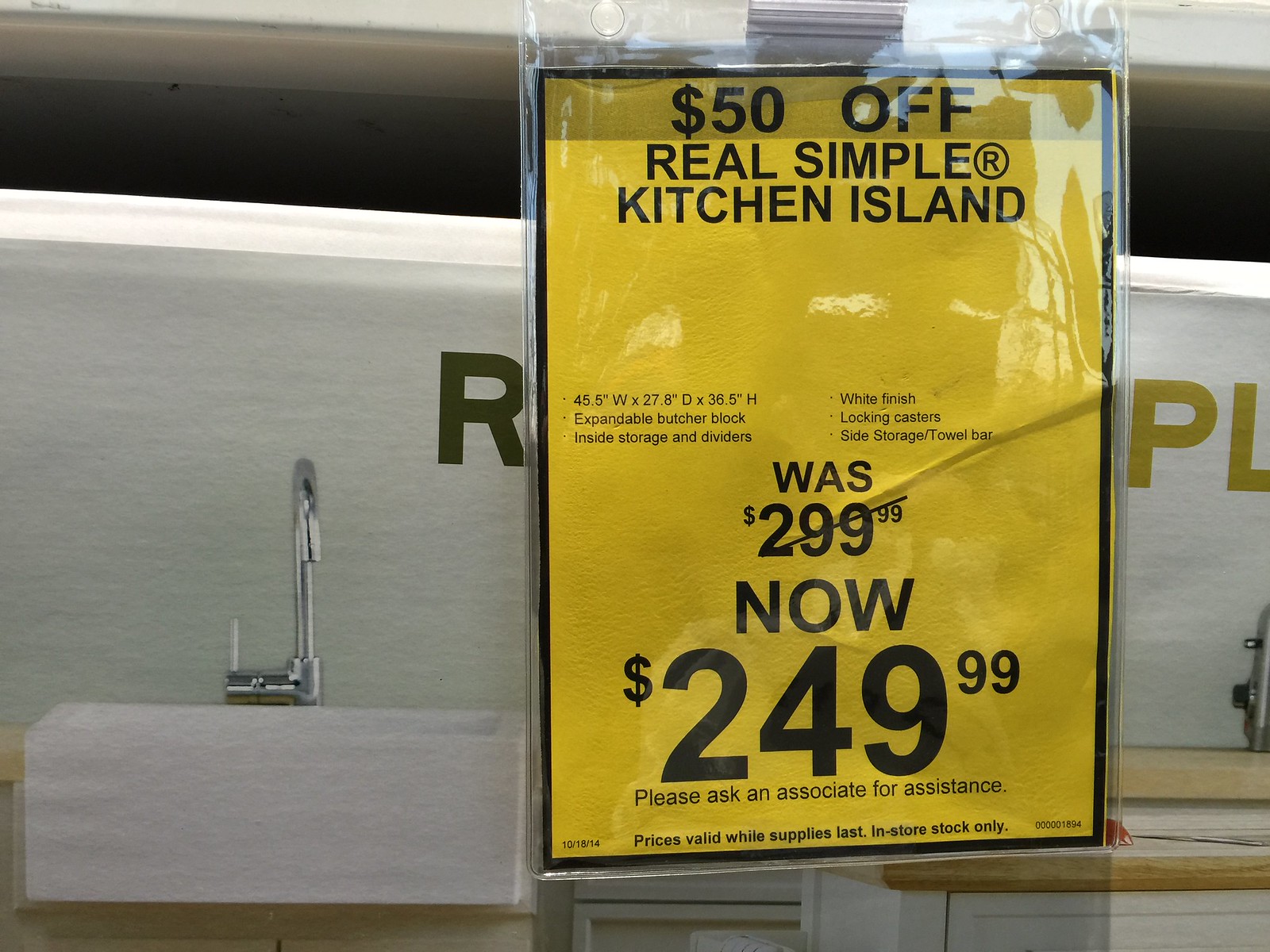This color photograph, likely taken inside a home improvement store like Lowe's or Home Depot, captures a close-up of a yellow price tag encased in a translucent plastic bag. The tag prominently advertises a $50 discount on a "Real Simple Kitchen Island", reducing its price from $299 to $249.99. The tag details the island's features, noting dimensions of 45.5" wide by 27" in diameter by 36.5" in height, and specifies a white finish with locking casters, a side storage towel bar, and an exchangeable butcher block inside storage and dividers. The sign advises customers to ask an associate for assistance, noting that prices are valid only while supplies last and for in-store stock only. In the background, the setting includes other items for sale, possibly sinks with linear designs and arched faucets, further suggesting a retail scene focused on home installations.